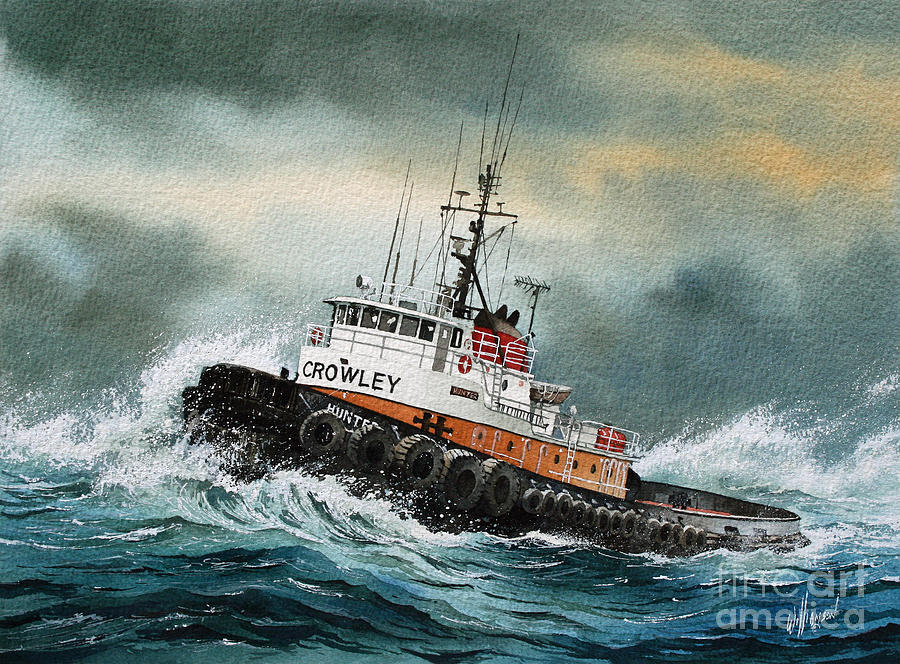This is a digital screenshot of a highly detailed painting depicting a tugboat named "Hunter" battling a fierce storm. The tugboat is the central focus and prominently features the word "Crowley" painted on the front of the bridge. The lower part of the vessel is painted black near the waterline, and it’s protected by side-by-side inflated tires of various sizes. The upper sections of the boat are orange and white, equipped with several ladders, railings, and antennas protruding from the bridge area. The stormy sky is painted in shades of gray with a brownish tint, intensifying the painting’s dramatic atmosphere. The restless sea beneath the tugboat is characterized by angry, white-capped waves, crashing and spraying around the vessel in vibrant blue tones, reflecting the chaotic environment. The painting captures the essence of the tugboat bravely navigating through the tempestuous waters without any visible crew, creating a tense and gripping visual narrative.